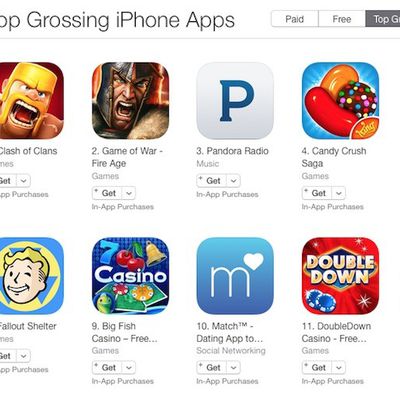This image, taken as a computer screenshot, showcases a display of mobile app icons organized into two horizontal rows, with four icons in each row. At the top left corner of the screenshot, partially obscured text can be seen which reads something about "grossing phone apps." The categories "paid," "free," and partly obscured "top" are also visible.

On the top row, the first icon from the left features a cartoonish image of a guy screaming. The second icon is similar, also depicting a cartoonish screaming character. The third icon is a simple blue "P" on a white background. The fourth icon presents orange and red jelly beans within a brown circle adorned with colorful dots, set against a blue background.

Turning to the bottom row, the first icon on the left displays a person's face with white skin and blonde hair against a blue and yellow background. The next icon to the right features the word "casino" with a blue seven, a red cherry, a bell, and playing cards along with red and yellow tokens. The following icon is a white "M" with a small white heart in its top right corner, set against a blue background. The final icon on the right of the bottom row has a red background and shows a blue diamond shape with a yellow outline, with the words "double down" in yellow text above it. Each icon has accompanying text beneath them, although it is too small to be entirely legible in the image.